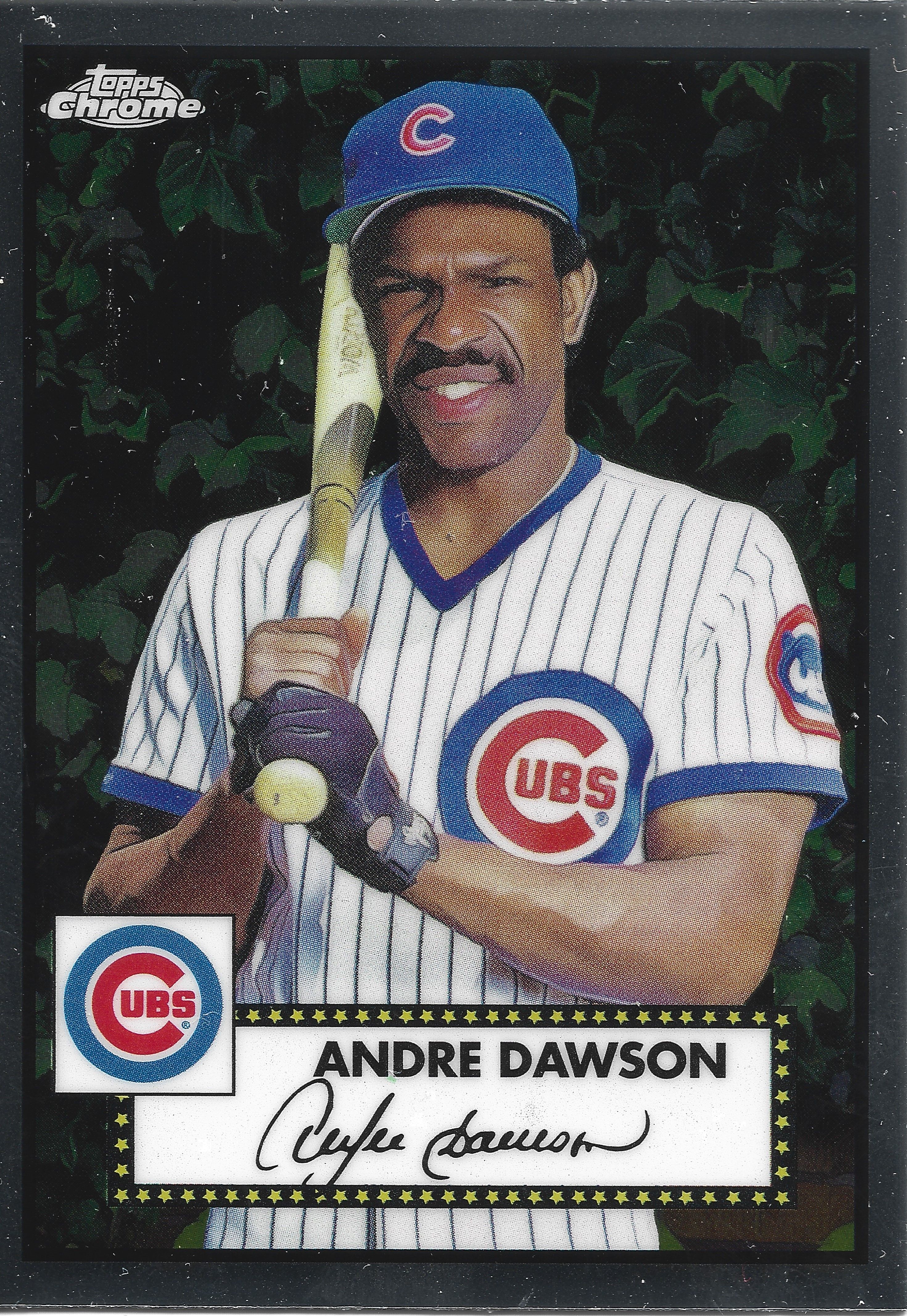This vintage baseball card is a Topps Chrome trading card featuring Andre Dawson, the legendary African American player for the Chicago Cubs. In this full-frame image, Dawson is shown in his classic Cubs uniform, which is white with vertical black stripes and features darker blue accents around the sleeve and V-neck. A prominent red "Cubs" logo inside a circle is displayed on his chest. He sports the team's blue baseball cap, emblazoned with a red "C" outlined in white. Andre Dawson poses with a baseball bat resting on his left shoulder, gripping it with his right hand, which is clad in a single black glove. He gazes directly at the camera with a neutral expression against a backdrop of lush green ivy, indicative of Wrigley Field. The bottom of the card features a white rectangle bordered by black and yellow stars, displaying "Andre Dawson" in black print and his signature in black cursive below it. The Cubs logo is situated next to his name, similarly enclosed in a box with a black outline. The entire card is framed by a gray border, adding to its classic aesthetic.